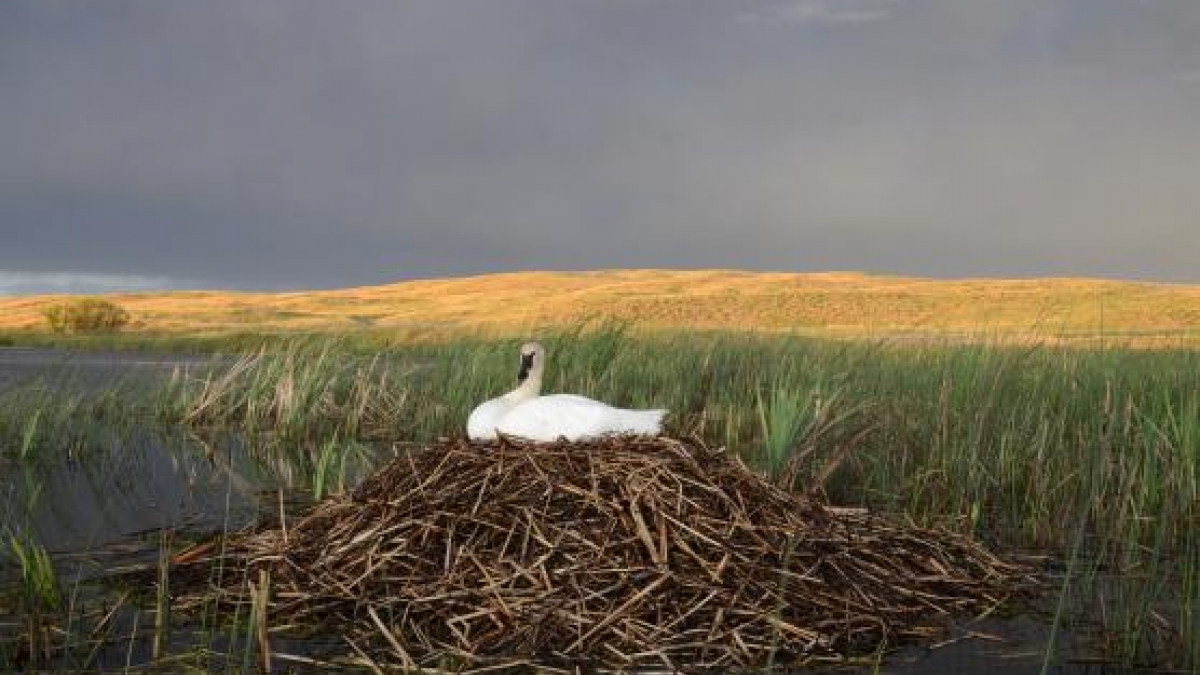A beautiful and detailed photograph captures a lone swan perched regally on a large nest made of sticks and dead grasses, situated in a marshy area. The scene is set in what resembles a Norwegian fjord, devoid of trees but rich with reeds and seagrasses. In the background, a yellow grassy hill stretches into the distance, suggesting late summer or autumn, with the sky above filled with ominous gray clouds hinting at an impending storm. The swan's pure white feathers stand in stark contrast to the dark, moody landscape, adding to the image's striking visual impact. Although the image appears to be of lower fidelity, making fine details hard to discern, the multi-layered composition and the swan's solitary presence evoke a sense of tranquility and isolation.